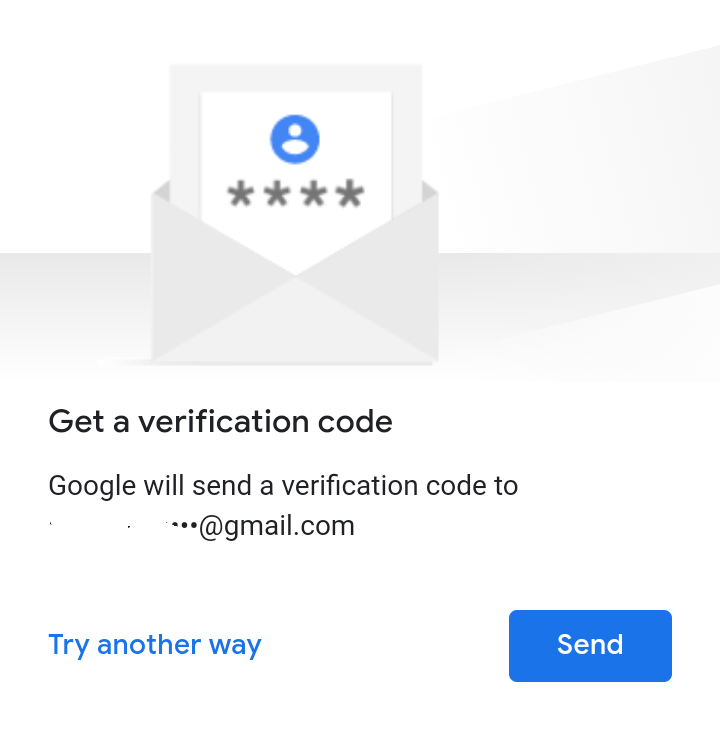The image showcases a Gmail notification. At the center of the notification is an envelope icon, partially opened to reveal a message. Within the message, there is a placeholder for the user's profile photo, represented by a gray circle, followed by four asterisks, symbolizing a partially obscured email address. Below the envelope graphic, the text reads "Get a verification code." Further down, the message specifies, "Google will send a verification code to," followed by an ellipsis and "@gmail.com" to indicate the partially hidden email address for security purposes.

Additionally, beneath this instruction, in blue text, are the options "Try another way," offering alternative verification methods, and a prominent "Send" button to initiate the code-sending process. This detailed Gmail notification clearly guides the user through the steps to receive a verification code for secure access.